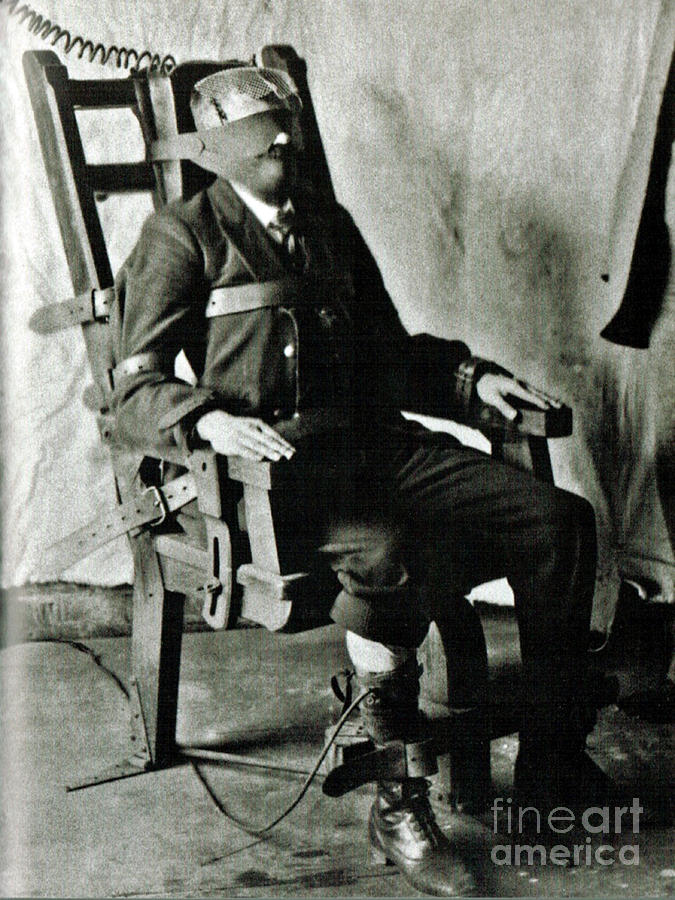The image depicts a very disturbing black and white photograph of a man strapped into an electric chair, likely dating from the early 20th century. This grim scene shows the man wearing a dark suit with a white shirt and a tie, indicating he is dressed formally. His face is mostly obscured by a leather mask that holds his head against the chair's back, with only his nose visible through a cutout. The man’s wrists, chest, waist, and ankles are tightly secured with thick belts, and a coiled wire runs to his head, suggesting the imminent execution. Additionally, electrodes are attached to at least one of his feet. The large wooden chair he is strapped to has open box-like structures behind it, adding to the menacing aura. The background features a hanging canvas cloth, and the floor beneath the chair appears dirty and worn. In the lower right corner, there is a watermark attributing the photograph to Fine Art America. Overall, this is a clear and well-lit image, providing a stark and haunting portrayal of the scene.